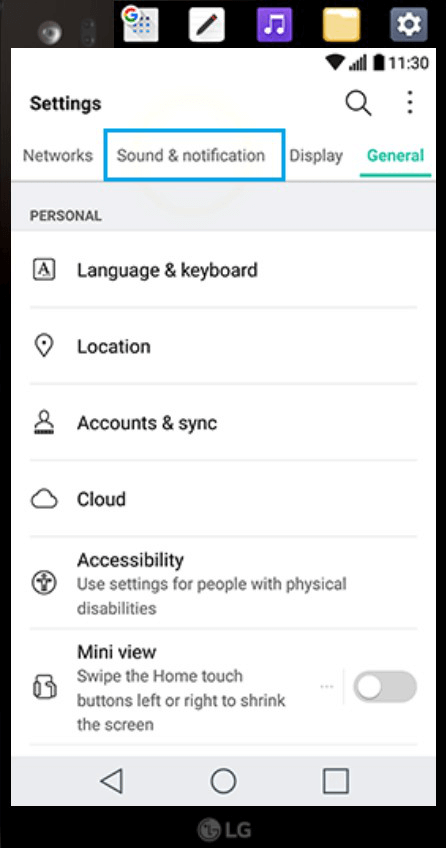A detailed screenshot of a cell phone's settings menu is displayed. The top section features essential status indicators including the reception cell phone signal icon, a low Wi-Fi signal icon, a battery icon, and the time, which reads 11:30, all aligned on the upper right-hand corner of the screen.

Below the status indicators, the word "Settings" appears prominently to the left. The main settings interface is divided into four tabs: "Networks," "Sound & notification," "Display," and "General." The "Sound & notification" tab is emphasized with a blue box surrounding it, indicating it is currently selected. 

The "General" tab is highlighted with green font, suggesting that it is the active section being viewed. Under this "General" section, the title "Personal" is listed first. Following this title are various settings options: 

- "Language & keyboard"
- "Location"
- "Accounts & sync"
- "Cloud"

Further down, an "Accessibility" option is listed for adjusting accessibility features. Lastly, the "Mini view" setting is visible, equipped with a toggle switch that is currently set to the off position.

The careful layout and clear labeling on this screenshot provide an organized view of the phone's settings, facilitating easy navigation for users.